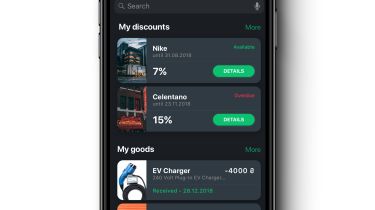A small vertical image appears to be a screenshot taken from a smartphone. The phone is positioned against a white background, with a subtle gray shadow creating a gradient effect fading out to the white, accentuating the right-hand side. The smartphone itself is black at the top, featuring a gray bar with a search field. On the left-hand side of this bar is a magnifying glass icon, and on the far right is a microphone icon, indicating voice search functionality.

Below the search bar, the background is black and prominently displays the text "My Discounts" in white. A green "More" button is visible beneath this title. Two rounded rectangular gray boxes, each with a picture icon, are lined up vertically beneath this section. The first box contains the word "Nike" above smaller gray text that reads "7% More". There is a green, although blurry, button labeled "Details" adjacent to it.

The second box is slightly more challenging to discern but seems to feature the word "Selen Tano," accompanied by an indication of a 15% discount, noted in red text. This also includes a green "Details" button. Following this section, the text "My Goods" appears, relating to an EV charger listed with a discount of around $4,000 and additional information specifics.